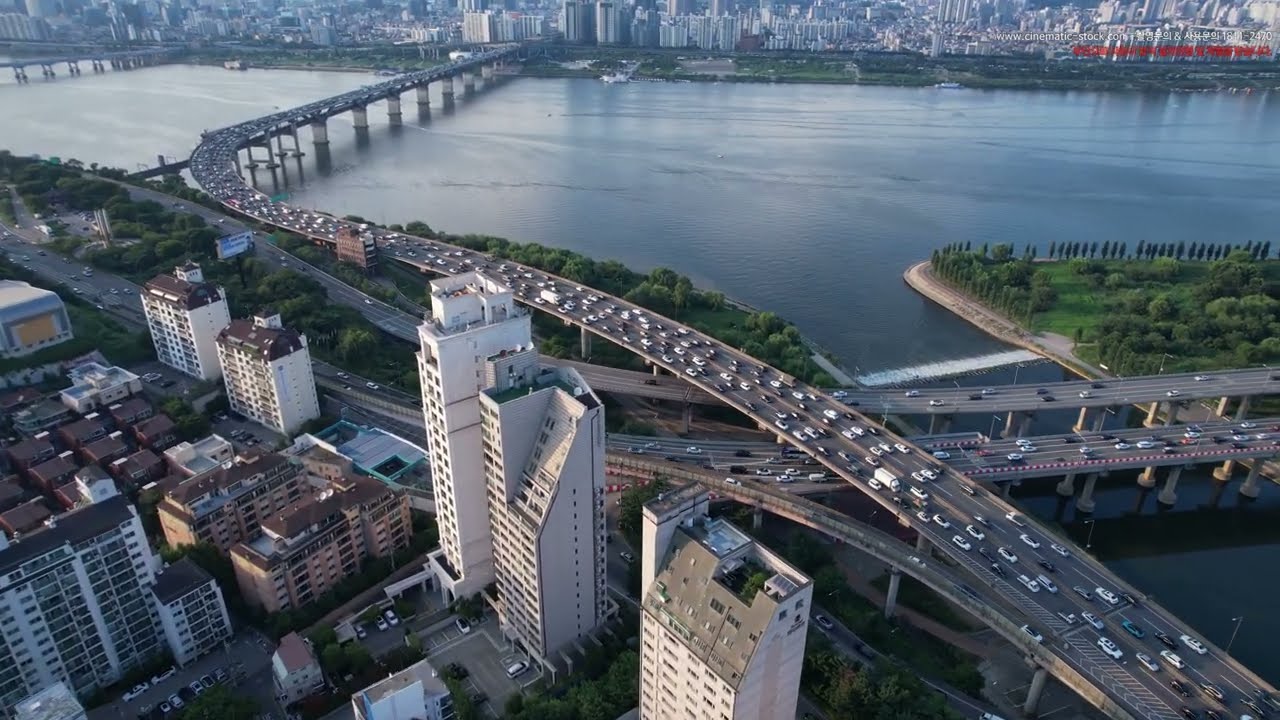This is an overhead daytime photograph of a bustling urban area. The image likely taken from a high vantage point such as a drone or helicopter, capturing the intricate layout of a city divided by a large, still body of water, possibly a river or harbor. On the top right of the image, there is a watermark from cinematicstock.com with some red lettering and symbols underneath it. 

Dominating the scene is a multi-lane freeway, heavily congested with vehicles, which starts from the lower right-hand corner and curves towards the top center of the image. This busy roadway crosses the body of water via a prominent bridge. Another bridge can be seen in the top left corner of the photograph, also spanning the water. 

The foreground and background are filled with a dense array of tall buildings, indicative of a high-rise, metropolitan environment. To the left side, near the bottom, multiple multi-story buildings with numerous windows and possibly car parks are visible. The right side of the image shows roadways running parallel to the shoreline, interspersed with patches of greenery, including some parkland. The overall scene is marked by a striking contrast between the urban infrastructure and occasional green spaces, encapsulating the essence of bustling city life.